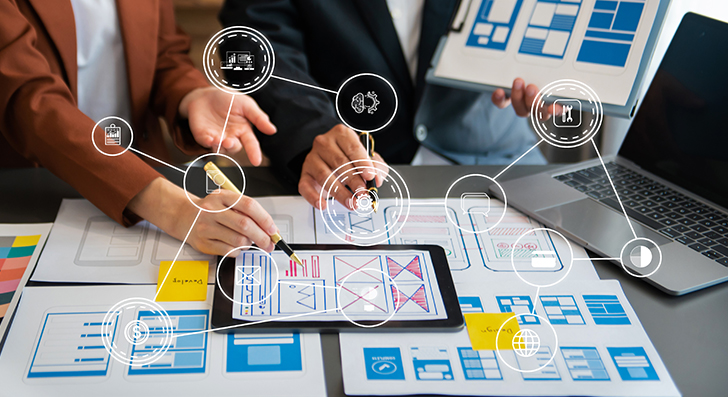This image is a stock photograph depicting a focused work meeting between two individuals. Both are standing over a table, engrossed in a detailed technical discussion. The man on the right, dressed in a blue suit, holds a pencil in his hand, while the woman on the left, wearing a cinnamon-colored coat with a white blouse, points to a design displayed on an iPad. The iPad, which appears to be about the size of an 8 1⁄2 by 11 sheet of paper, rests on a surface cluttered with various blue and white schematics, likely representing app or menu system designs and flowcharts. Additionally, in the background, another hand holding a clipboard with similar blue-and-white drawings is visible. A laptop is positioned on the right side of the table. Overlaying the entire scene are digitally added circles connected by lines, suggesting relationships between concepts or elements, including one with a dollar sign, indicating financial aspects. The overall setup appears to demonstrate or plan an engineering or business process flow.